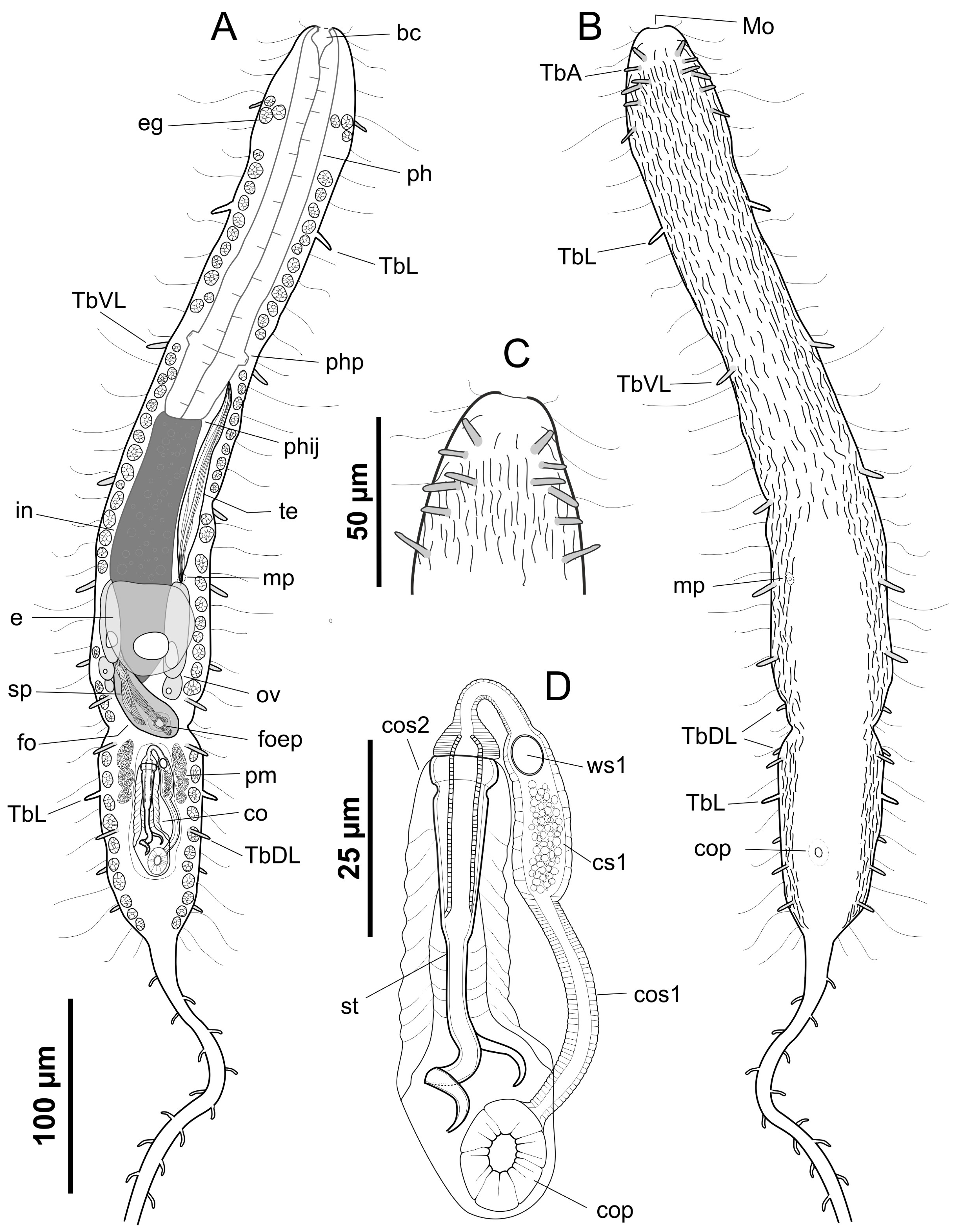The image is a highly detailed, black-and-white scientific diagram composed of four main sections labeled A, B, C, and D. Label A depicts a structure resembling a snake or plant pincher with hairs along its sides and spikes on its tail, extending to a measurement marker indicating "100 μm." The top view of this structure is shown in Label B, providing a different perspective. Label C highlights the head of the structure observed in both A and B, offering a close-up look. Label D illustrates the internal cross-section of the structure, revealing its intricate inner workings and cellular composition. The diagram appears to feature fibrous textures and possibly reproductive elements, such as an egg sac, demonstrating a high level of detail in what seems to be a zoomed-in representation of a plant or similar organic entity.